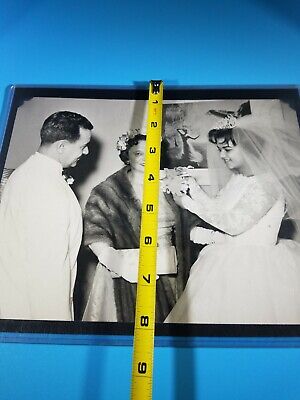This is a detailed black and white photograph of a wedding scene, laid on a light blue table. The image, framed in black, is approximately 8 to 10 inches long, as indicated by a yellow measuring tape stretched across its center. In the photograph, three people are prominently featured: the bride, the groom, and a woman who appears to be one of their mothers.

The groom, standing on the left, is dressed in an all-white suit with a long coat and a boutonniere. He has dark hair and looks directly at what the bride is holding. The bride, positioned on the right, wears a beautiful white wedding gown and a pretty veil that flows behind her head, revealing her face. She has black hair and holds an object in her hand. Central to the image is an elegantly dressed woman, presumably a mother, adorned with a fur stole draped over her dress. She has flowers either in her hair or hat, adding to her sophisticated appearance.

In the backdrop of the black and white photo, there is another picture depicting a woman wearing a dress with a hand on her head. The measuring tape across the photo suggests precise attention to detail, enhancing the composition's observational nature.